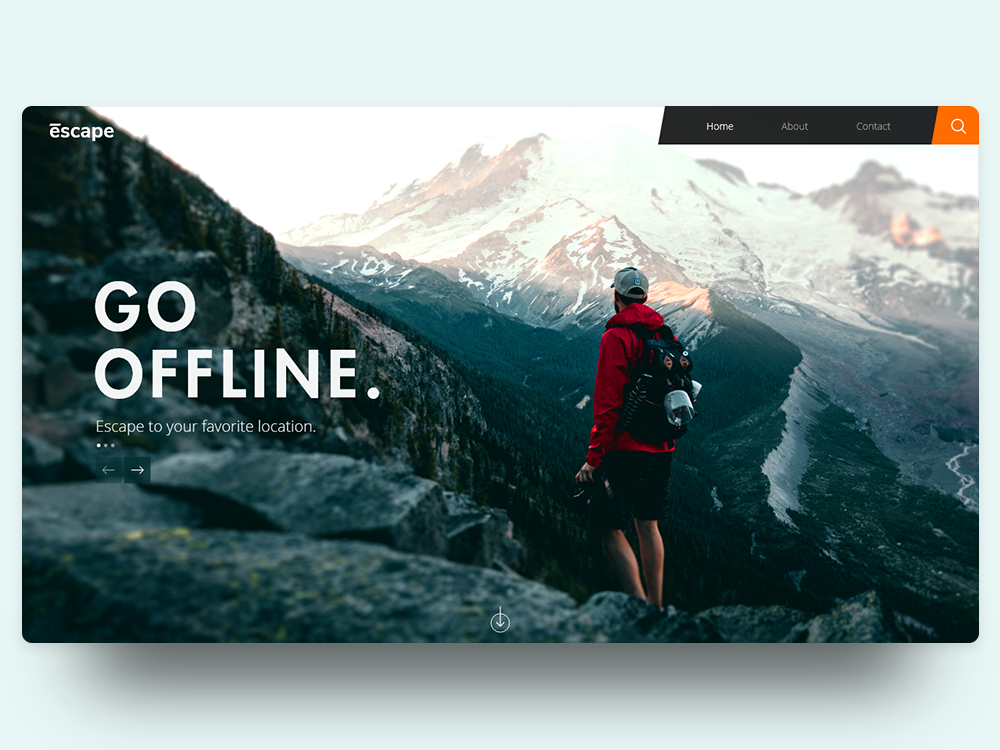The website's homepage features a stunning image designed to evoke a sense of adventure and tranquility. In the upper left-hand corner, the site's name, "escape," is written in lowercase letters with a distinctive line above the "E." On the upper right side, a search bar and other navigation elements are present. 

Dominating the center of the image is an inspirational tagline, "Go offline, escape to your favorite location," inviting visitors to disconnect and explore nature. The background showcases a breathtaking landscape of multiple snow-capped mountain peaks, with one prominent peak directly ahead. The mountains are partially covered with snow, revealing rocky, untouched sections.

In the foreground stands a lone hiker, equipped with a backpack and wearing a hat, a red hoodie, and black shorts. He stands on a separate mountain, gazing out over the vast, rugged terrain that stretches before him. The view includes a series of caverns between the foreground mountain and those in the distance. To the right, the landscape drops sharply, suggesting a steep and dramatic descent. The entire scene paints a picture of serene wilderness and the exhilarating potential of outdoor exploration.